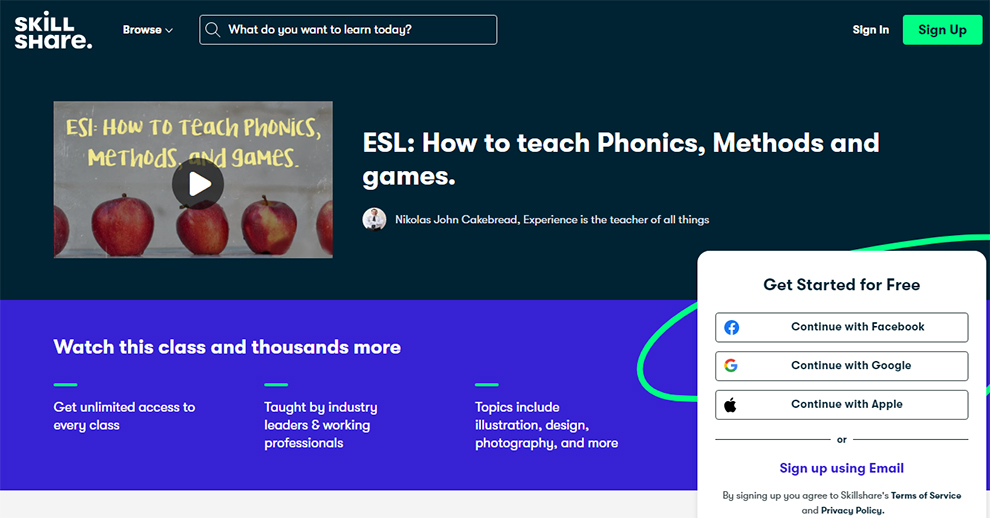On this webpage, we see the layout of the Skillshare website, a platform designed for individuals to create and sell courses or to enroll in them. The main page features a dual-color scheme of dark blue and light green-turquoise, which helps differentiate various sections. Below this, there's a section in a more classical blue color.

At the top of the page is a search bar for browsing courses, along with a sign-up/sign-in option located in the top right corner. The sign-up button stands out in light green-turquoise. Just below the search bar is a video thumbnail displaying a row of apples with yellow glittering text that reads, "ESI: How to Use Phonics Methods in Games." This course is created by Nicholas Jean Cakebeard, described as an experienced teacher in various topics.

The homepage also provides additional details, such as how to navigate the website, the topics it offers, and the instructors available. At the bottom right corner, there's a "Get Started for Free" bar, which allows users to log in via Facebook, Google, or Apple, or sign up using their email.